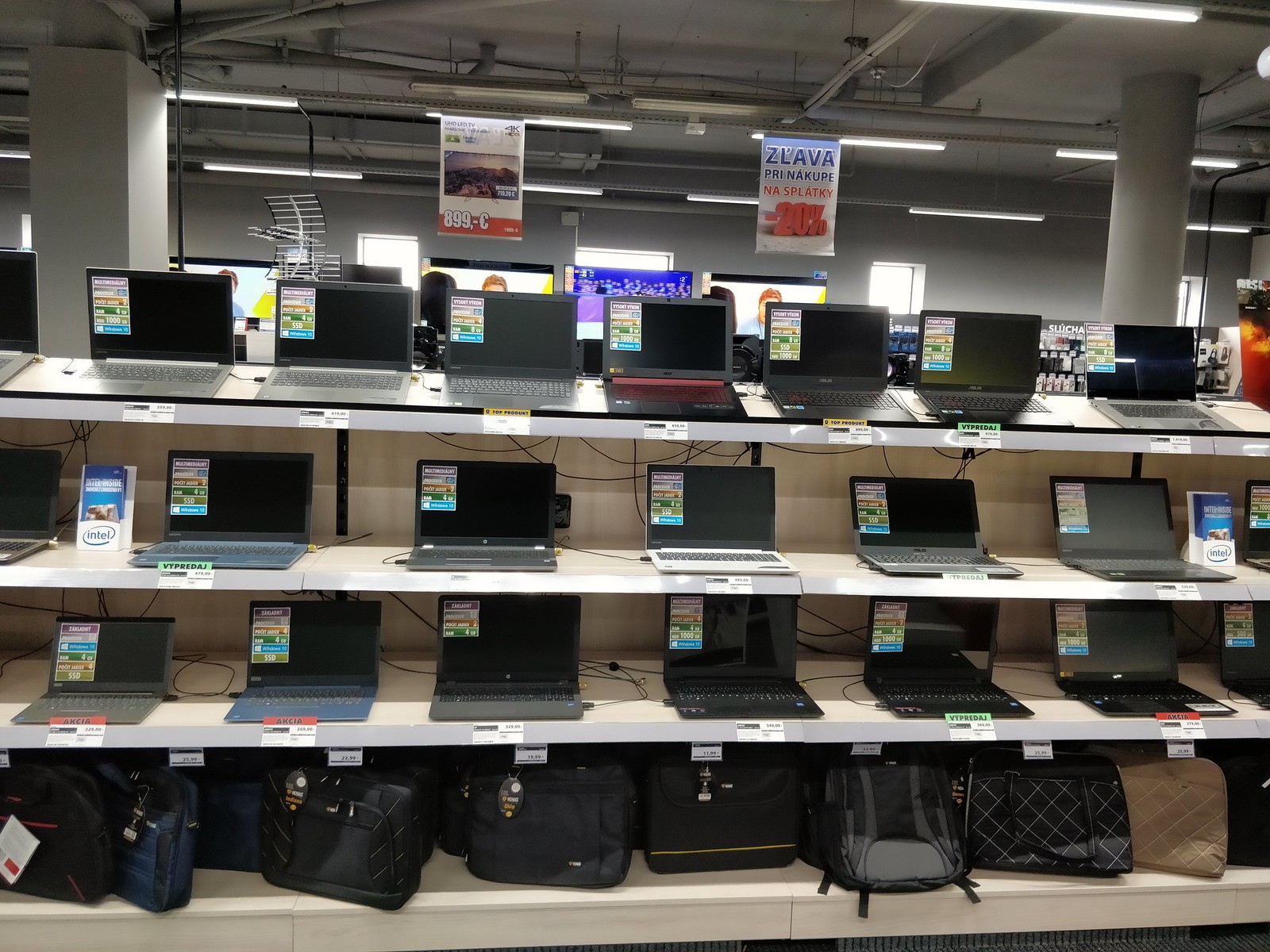This detailed photograph depicts the interior of an electronics store specializing in computers. At the center of the image is a prominent shelving unit with four levels, all lined up with various electronics. 

The bottom shelf prominently displays a variety of computer cases standing upright, mostly black with the exception of one tan bag. The shelves above—specifically the second, third, and fourth tiers—feature an array of laptop computers arranged side-by-side with their screens open. Each laptop is accompanied by informational stickers detailing specifications and price tags displayed in front.

The shelving unit itself is noteworthy, consisting of white surfaces with a light tan background. The store ambiance is industrial, characterized by an exposed ceiling with visible pipes and fluorescent tube lighting. Hanging from the ceiling are banners, one of which appears to offer a 20% discount while another advertises a screen or monitor priced at €899. Additionally, parts of other monitors and possibly TVs are visible further into the store, contributing to the tech-laden environment.

Natural light filters in through four visible windows, casting an inviting light over the well-organized display and enhancing the visibility of product details, making this an inviting space for shoppers interested in electronics.